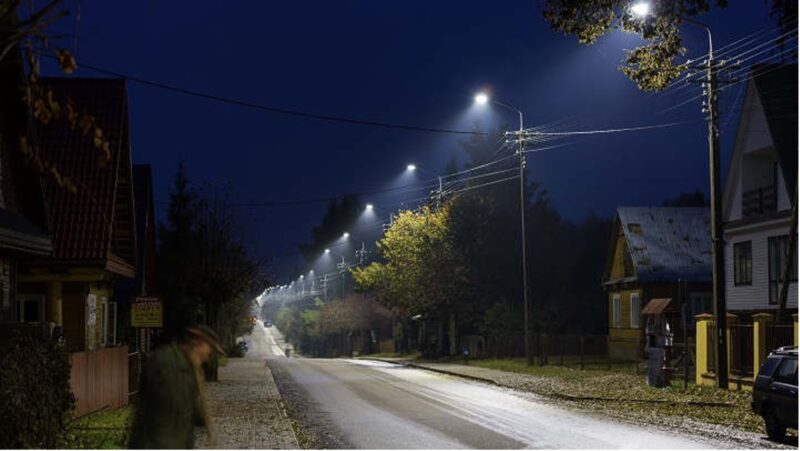This color photograph captures a tranquil suburban or rural street at night, under a dark blue, starless sky. The asphalt road runs through the middle of the image, flanked by cobblestone sidewalks. On the left side, there is a row of houses, one of which has a fence enclosing its yard, and a man walking into the frame in the lower-left corner. The right side showcases two houses initially, beyond which a line of trees and telephone poles with streetlamps stretches off into the distance. The street is illuminated by these evenly spaced streetlamps, casting a soft glow onto the road. A car is parked in the lower right-hand corner, and another is visible in the far distance. Leaves are scattered across the ground, adding to the autumnal ambiance. Additionally, a yellow, unreadable sign stands on a post to the left, completing this serene nighttime scene.